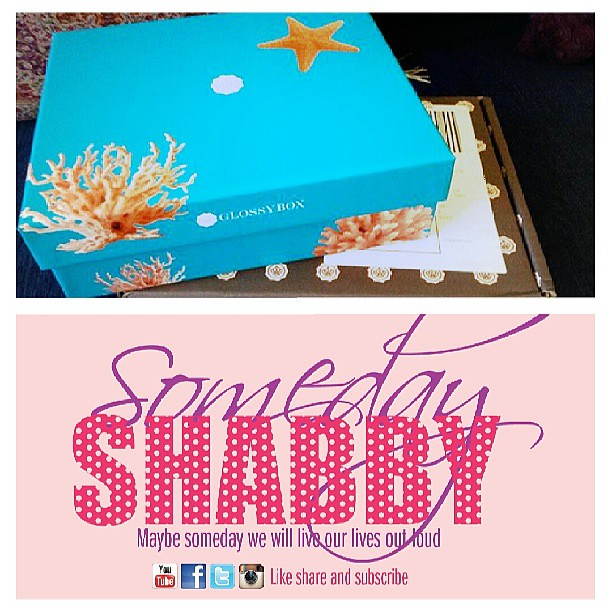In this detailed image, a blue box adorned with various sea-themed images, including corals and starfish, sits prominently at the top. The background is a stark black, providing a striking contrast to the colorful elements in the foreground. In the top-left corner, there is a fabric detail adding texture to the scene. The box, with "glossy box" text and logo centrally positioned, stands out clearly against the dark backdrop. Below this box, the bottom part of the image features a pink banner with the text "someday shabby" in a girly font, followed by the inspirational phrase "Maybe someday we will live our lives out loud." This section also includes social media icons for YouTube, Facebook, Tumblr, and Instagram, accompanied by the call-to-action "like, share, and subscribe." The colors throughout the image are vibrant and varied, featuring shades of pink, purple, dark pink, white, red, blue, light blue, brown, orange, and yellow. The composition suggests an advertisement for the "glossy box," with all elements arranged neatly and text easily readable.